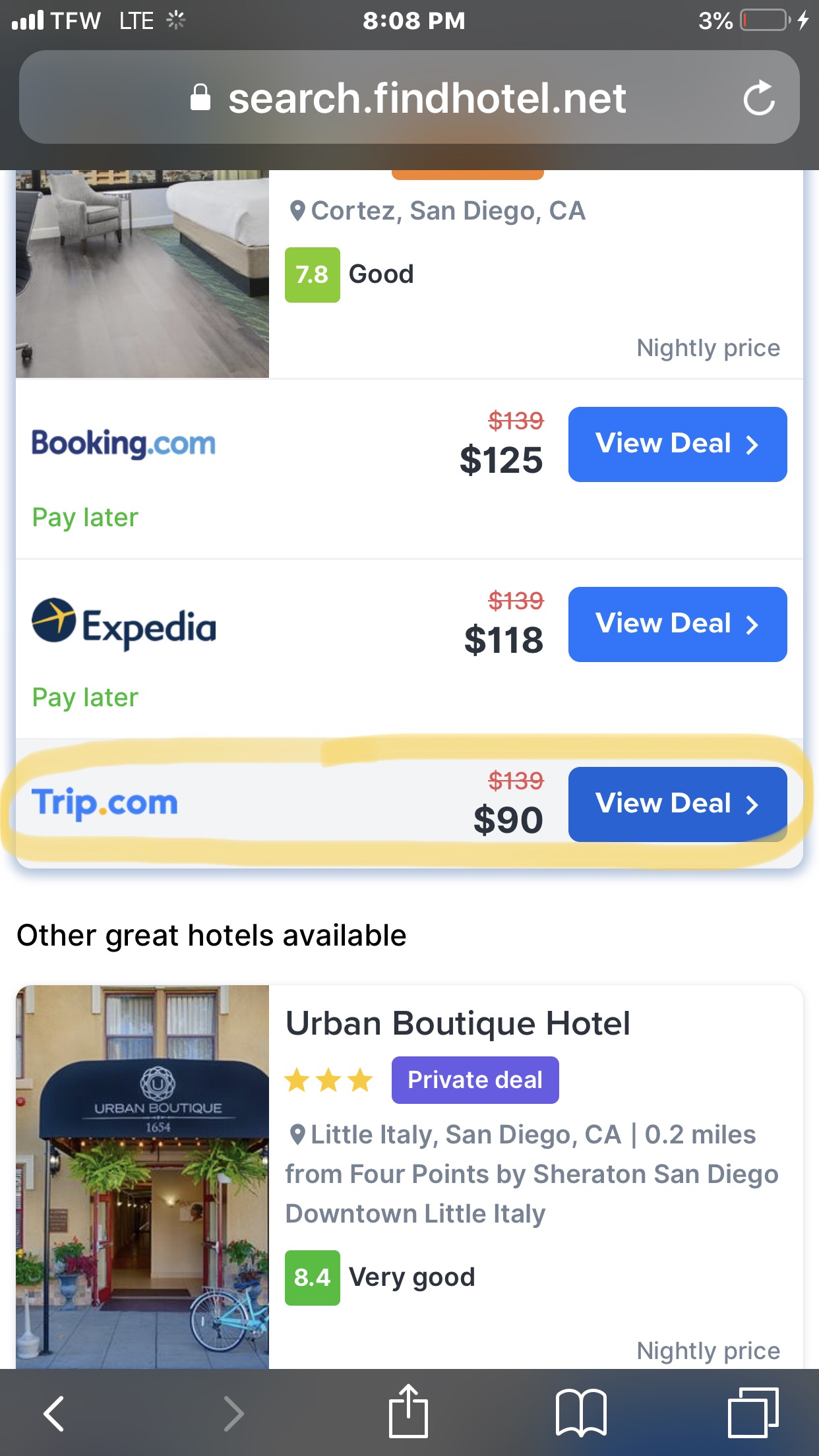The image is a cell phone screenshot from the website search.findhotel.net, which is clearly displayed in the web address bar at the top of the screen. Above this bar, the standard cell phone icons indicate the time and battery level. The website is currently searching for a hotel room in Cortez, San Diego, California, showing a property rated 7.8, indicating it is considered "Good."

Beneath this rating, three booking options are presented: Booking.com, Expedia, and Trip.com, with Trip.com listed last. Trip.com offers the most affordable rate at $90 per night, with a "View Deal" button situated to the right of this price. The next option, Expedia, lists a rate of $118 per night, and Booking.com shows the highest price at $125 per night. Following this section, there is an additional section titled "Other Great Hotels Available."

This detailed caption provides a comprehensive breakdown of the screenshot, highlighting the key information and layout of the webpage.